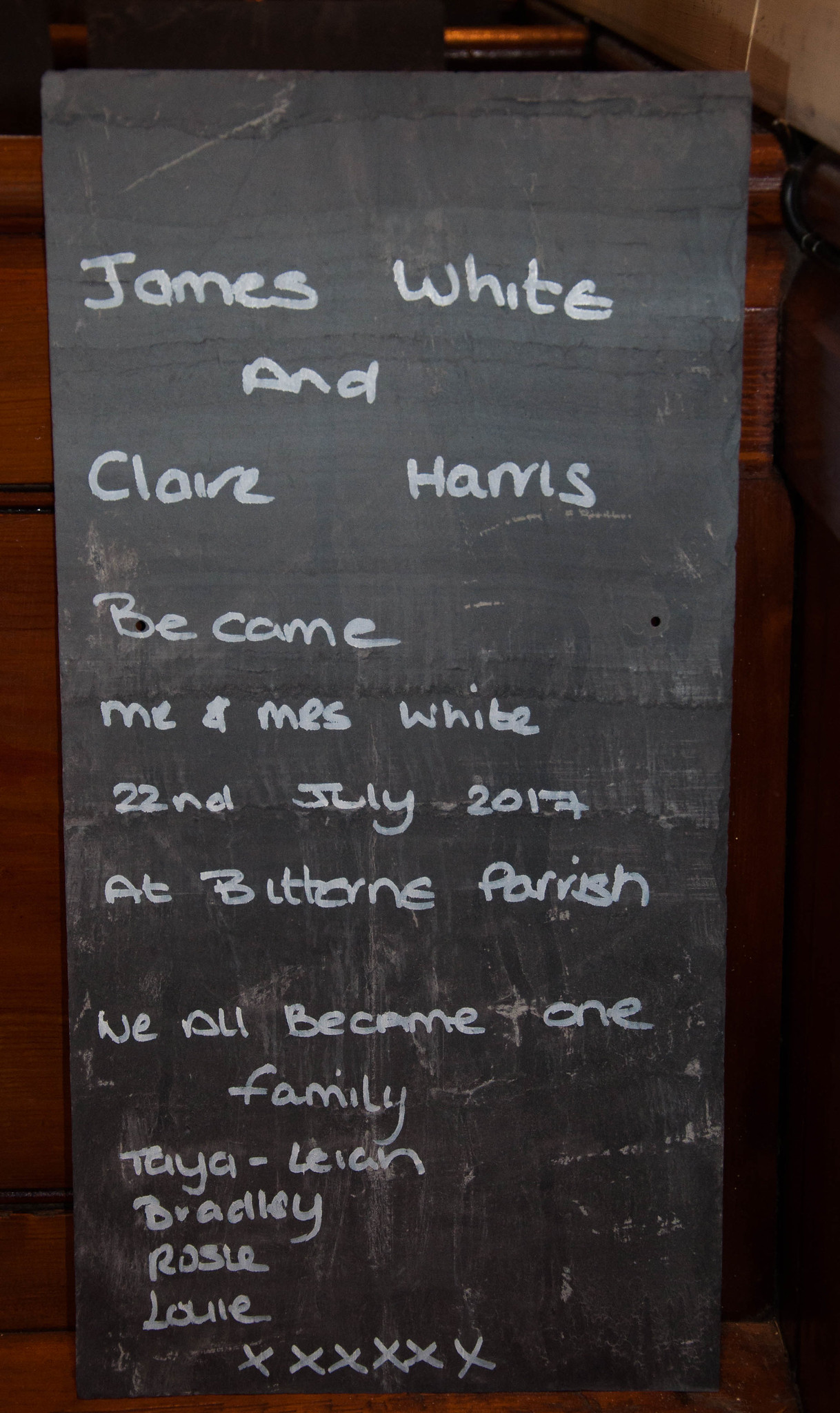This image captures a vertical rectangular black chalkboard with white chalk handwriting. It reads: "James White and Claire Harris became Mr. and Mrs. White, 22nd July, 2017, at Bittern Parish. We all became one family: Tanya, Leah, Bradley, Rosie, Lane." Six 'X' marks neatly line the bottom center. The chalkboard, appearing to be an indoor decorative sign, leans against a brown-colored wooden table, with a wooden floor visible in the background.